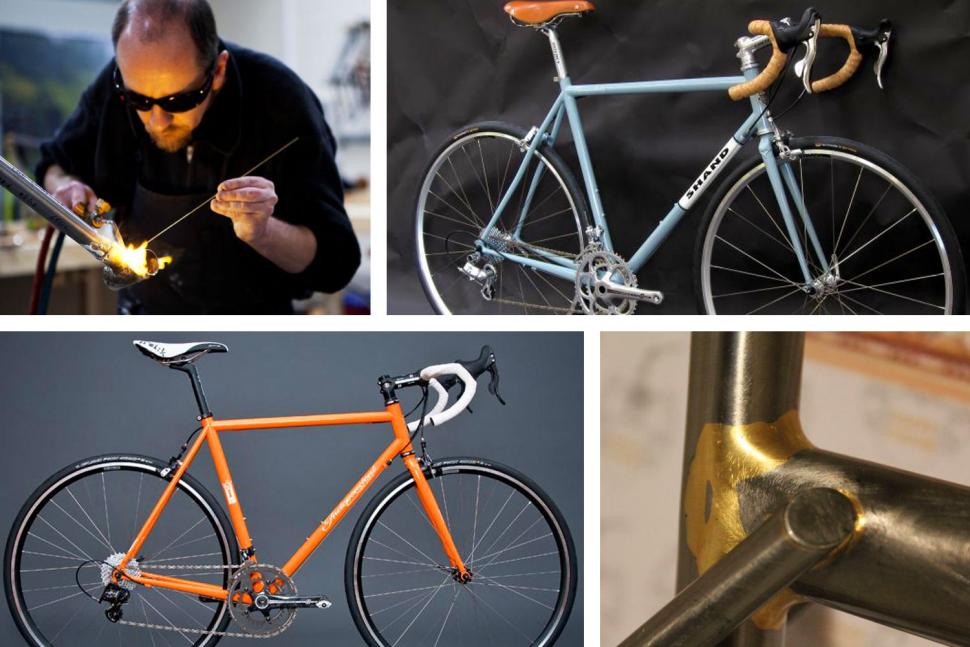This collage comprises four distinct photographs, meticulously arranged to create a cohesive rectangular image measuring approximately six inches wide by four inches tall. Each photograph showcases different stages and variations of bicycles, contributing to a unified theme. 

In the top left corner, a square photograph captures a man with light skin wearing sunglasses and a long-sleeve black shirt, welding a bicycle frame together with a welding iron. Adjacent to this image, the top right photograph displays a blue street bicycle gleaming with black tires, silver rims, an orange seat, and curved tan handlebars, set against a black background.

The bottom left corner presents another street bicycle, this time in vibrant orange. It mirrors the structure of the blue bicycle but features distinct details such as white handlebars and a white and black seat. Finally, the bottom right photograph offers an up-close view of a bicycle frame stripped of paint, showcasing the welds where one of the support rods has been attached to the main frame.

White border lines between each photograph crisply delineate the individual images, creating a visually organized and compelling representation of bicycle craftsmanship and design.